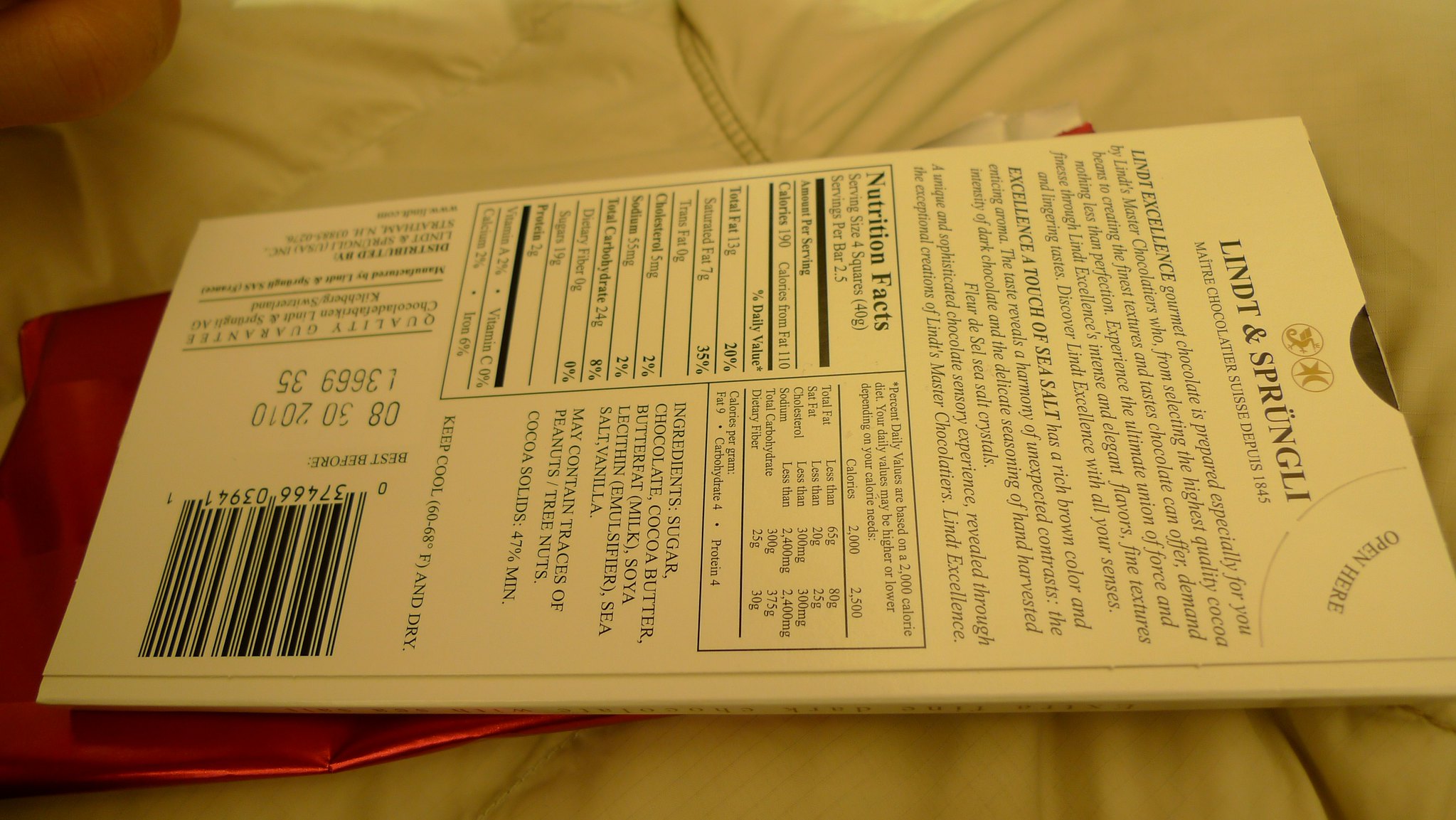This photograph captures the back of a candy bar package from the brand "Lindt & Sprüngli." The package features a detailed list of ingredients including sugar, chocolate, cocoa butter, butterfat, milk, soya lecithin (emulsifier), sea salt, and vanilla, with a note that it may contain traces of peanuts and tree nuts. The product boasts a cocoa solid content of 47% and highlights "an excellent touch of sea salt." The nutrition facts and other information are printed in very small letters. 

The candy bar's wrapper is displayed at an angle as if it was rotated to the right, requiring a tilt of the head to read the text clearly. The label also mentions an expiration date of October 30th, 2010. The packaging appears to be made from thin white cardboard with black lettering, and the chocolate itself is wrapped in bright pink foil. The package seems to be laid on someone's lap, possibly over a white jacket, adding a casual context to the image.